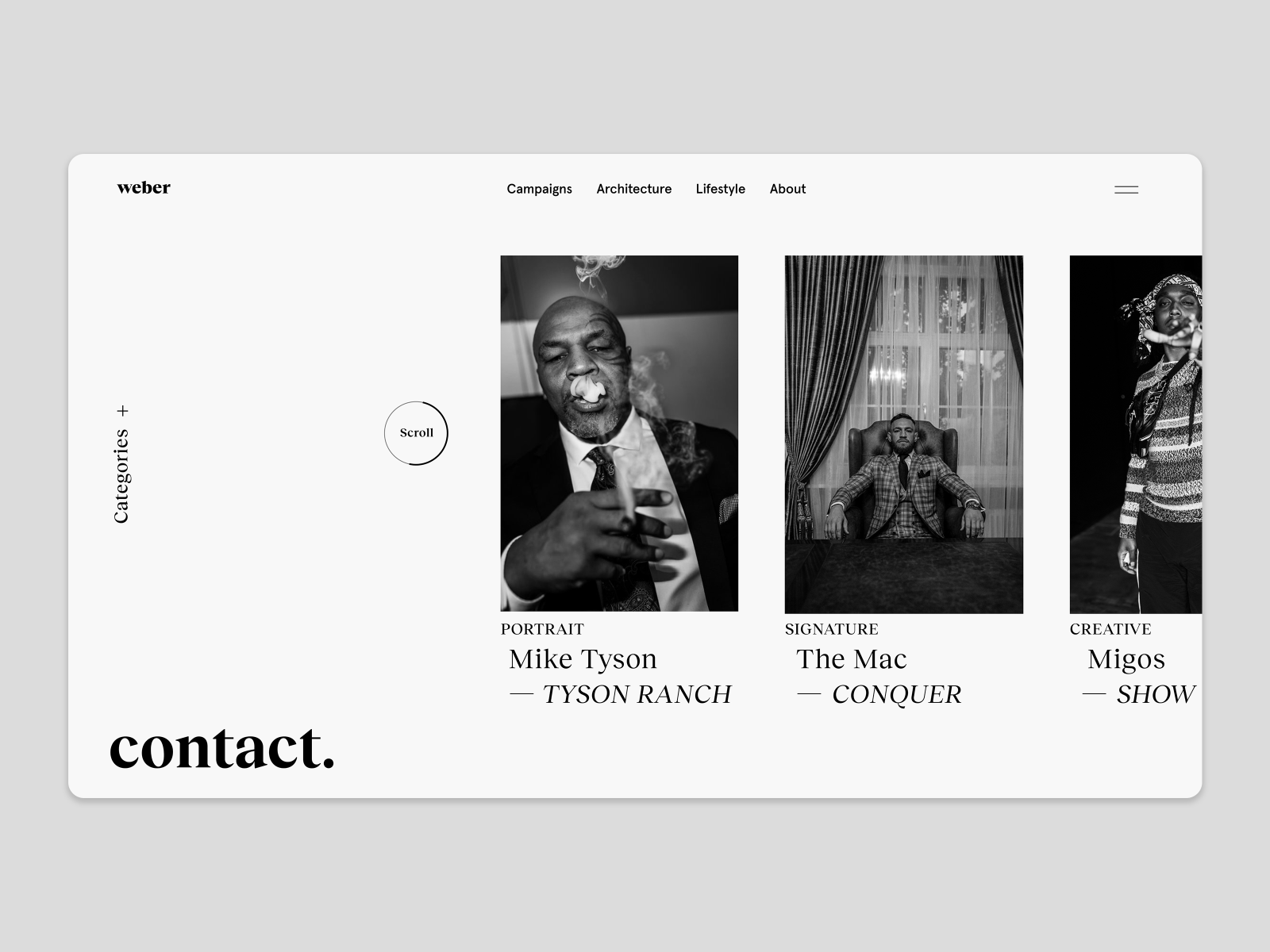The webpage, presumably belonging to a photography company named Weber, features a clean, white background adorned with black-and-white portraits of notable celebrities. The top-left corner prominently displays the name "Weber". The navigation menu at the top of the page includes sections labeled Campaigns, Architecture, Lifestyle, and About. 

Three striking photographs are showcased: 
1. Mike Tyson, impeccably dressed in a fancy suit, exudes charisma as he looks directly into the camera while smoking a cigar.
2. Conor McGregor, relaxed in a chair and clad in a suit, gazes confidently into the distance.
3. A member of the rap group Migos, donning a stylish sweater, stands with an air of casual elegance.

A contact button is positioned at the bottom left of the page, suggesting ease of reach for potential clients. The overall impression is of a sophisticated photography firm specializing in high-profile clientele.